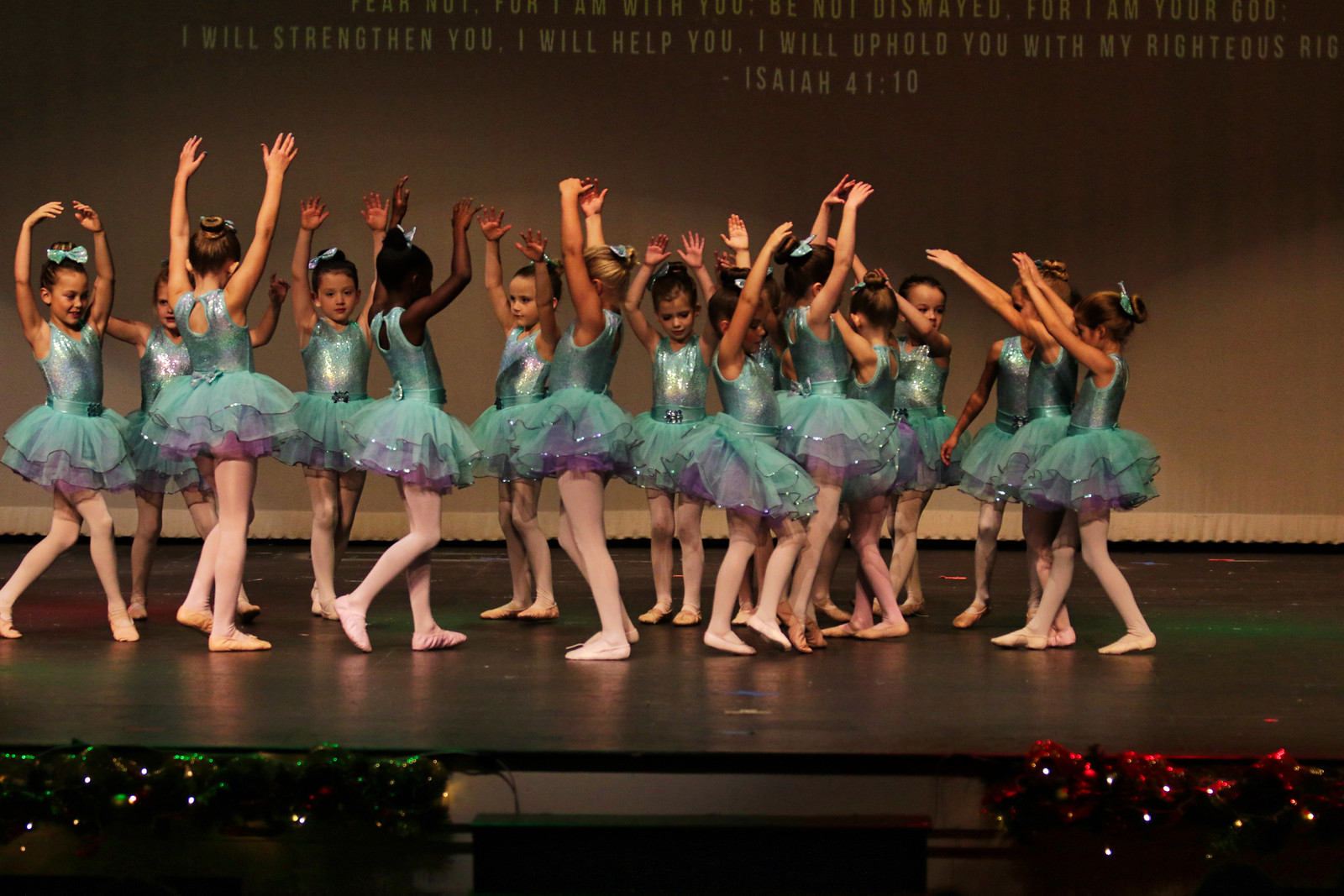In this vibrant photograph, at least a dozen young girls are performing a ballet dance on stage, each dressed in shimmering aqua green and purple tutus with matching green bows in their hair. They wear pink tights and ballet shoes, standing with their arms gracefully raised, facing various directions. The stage, with its brown wooden floor, is adorned with sparkling red and green garlands in front, suggesting a holiday performance, likely of a religious nature. The backdrop features a partially visible Bible quote from Isaiah 41:10, reading, "I will strengthen you, I will help you, I will uphold you with my righteous,” though some words are cut off. The overall scene is festive, joyful, and imbued with a sense of serene devotion.